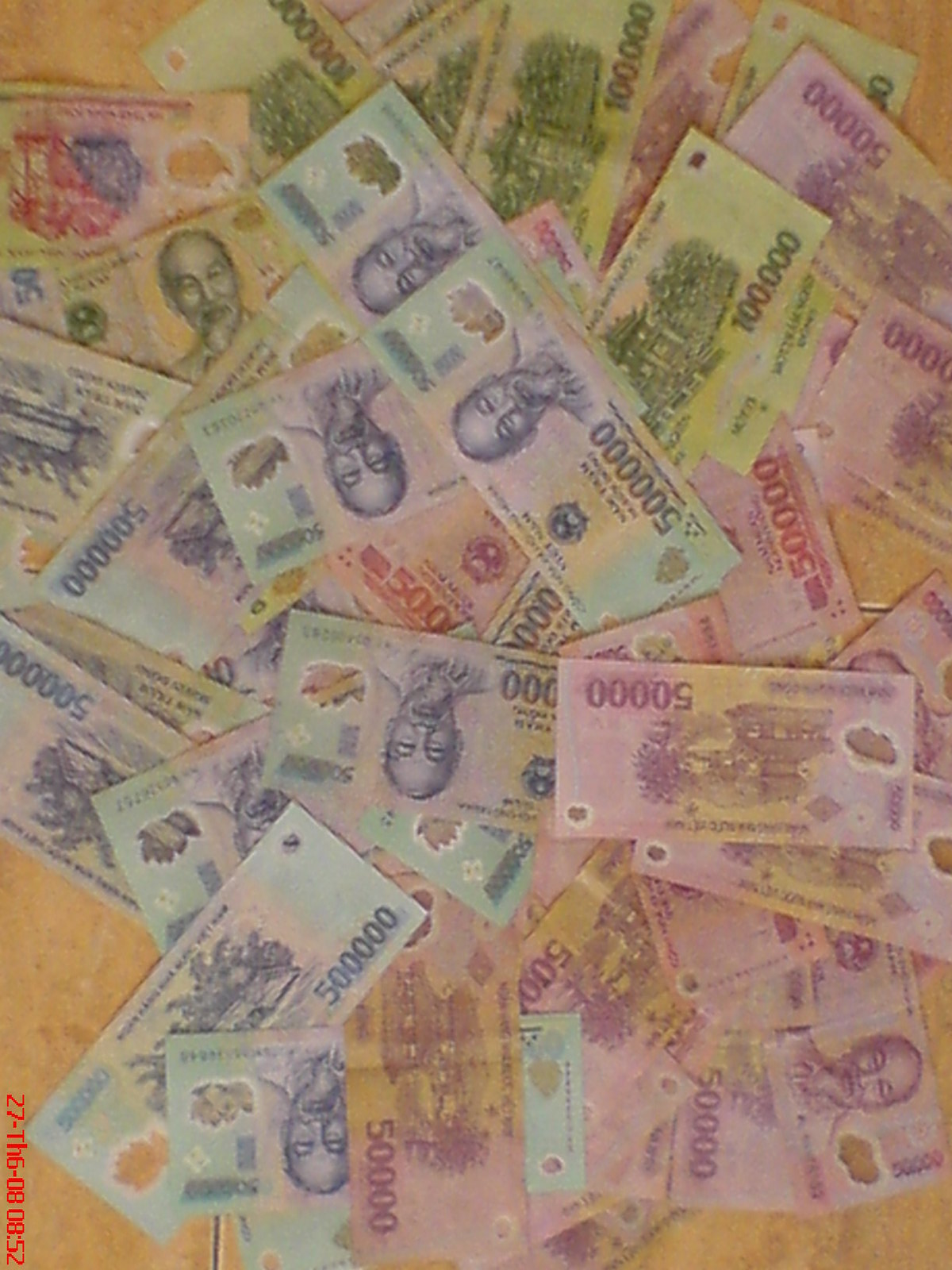This vertically aligned rectangular image showcases a collection of scattered currency on what appears to be a picnic table, easily identified by the dark separation lines between the wood slats at the bottom of the picture. The assorted paper bills are layered and positioned haphazardly across the brown surface, suggesting someone might have just dumped them out, possibly readying to count the total amount. The bills are vibrant in color, featuring hues of yellow, pink, green, purple, and blue. The yellow bills prominently display the figure 100,000 (or 100.000, depending on how it's read), while the purple and blue bills indicate amounts of 50,000 and 500, respectively. A distinct detail in the lower left-hand corner of the image is a red sideways print that reads "27-TH6-08-852." The varied currency denominations and colors create a visually rich and somewhat chaotic scene on the rustic table.